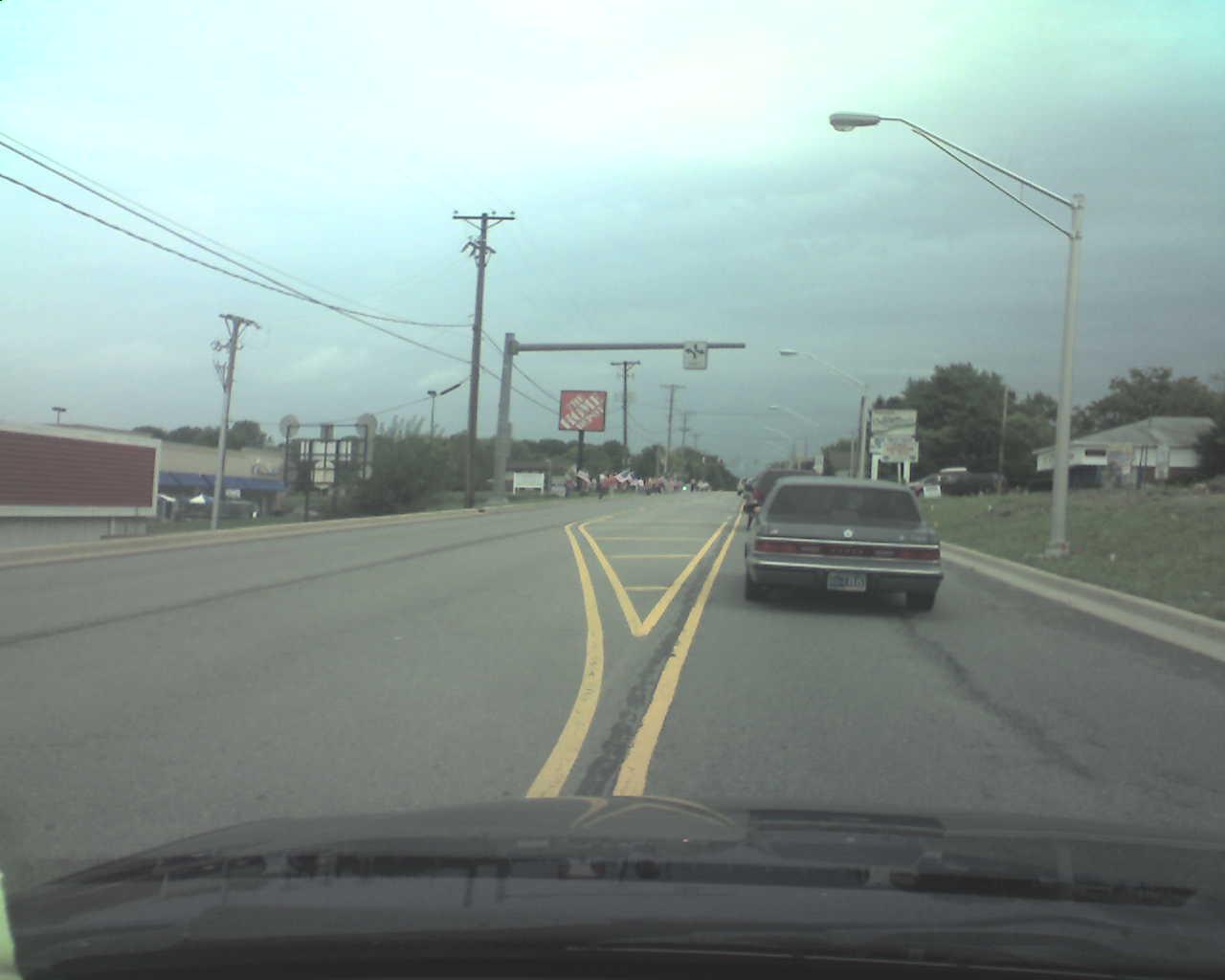A square-format photograph taken from inside a car showcases the vehicle's interior, capturing portions of the dashboard, windshield, and hood. The scene outside reveals the driver is traveling on a right-hand lane, demarcated by yellow center lines which indicate the opposing direction of the lane on the left. Directly ahead, another car is visible. On the right side of the road, a light pole bends over to illuminate the pathway. A green embankment flanks this side, suggesting grass or other vegetation. In the background, a building surrounded by trees is discernible. The left side of the image features more buildings, a telephone pole with wires stretching along the length of the road, and a prominent orange billboard with white text.